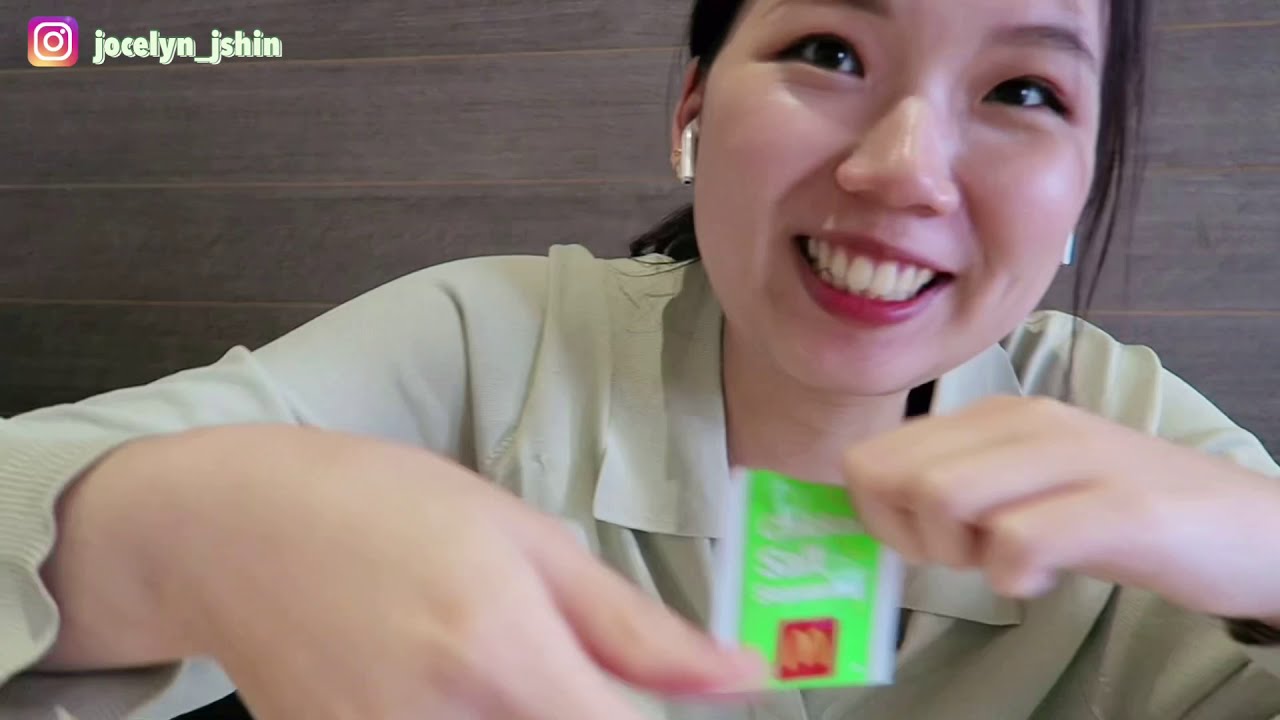In this Instagram screen grab, an Asian woman named Jocelyn is featured prominently in a video. The Instagram logo and her handle, "Jocelyn_JShin," are visible in the top left corner. Jocelyn is smiling warmly at the camera, giving an impression of happiness and engagement. She's wearing a pale green blouse and has Apple EarPods in her ears. Jocelyn is holding up a McDonald's sauce packet with a green and white label, likely a sweet and sour sauce, towards the camera, suggesting an unpacking video or a product feature. The background shows a wooden wall, indicating she might be inside a restaurant or a similar setting.